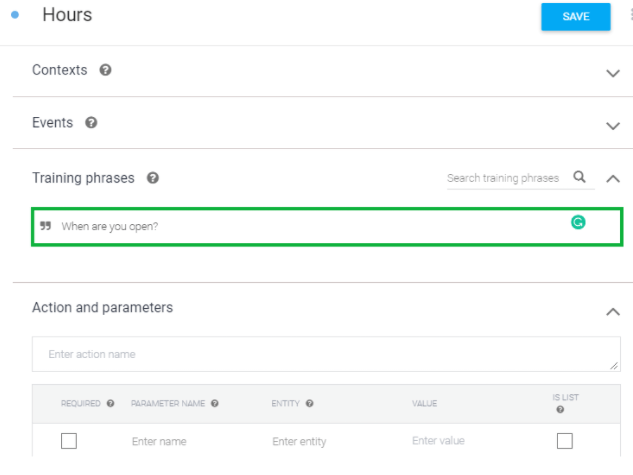This image is a screenshot of a user interface for an app or software program, featuring a clean, predominantly white background with various segmented sections delineated by gray lines. 

At the top left corner, the section labeled "Hours" is marked by a blue dot. Opposite this, on the right side, there's a blue button with white text that reads "Save". Below this, the next section begins with a gray line and is titled "Context" on the left. Adjacent to "Context" on the right is a down arrow, indicating a drop-down menu.

Continuing in this pattern, another gray line separates the next section labeled "Events" on the left, followed by "Training Phrases" which uniquely features a search box on the right. Underneath this, there's a large green highlighted box containing the phrase "What are you open?" suggesting it’s a key phrase within the training data.

Further down, after another gray line, there’s an "Action and Parameters" menu. This section includes a search box labeled "Interaction Name" and several input fields where users can specify details such as "Required", "Parameter Name", "Entity", "Value", and "List." Each input seems to allow for either typing or selection from predefined options.

The entire layout is structured for ease of use, with clear segmentation and interactive elements designed to streamline user interaction.